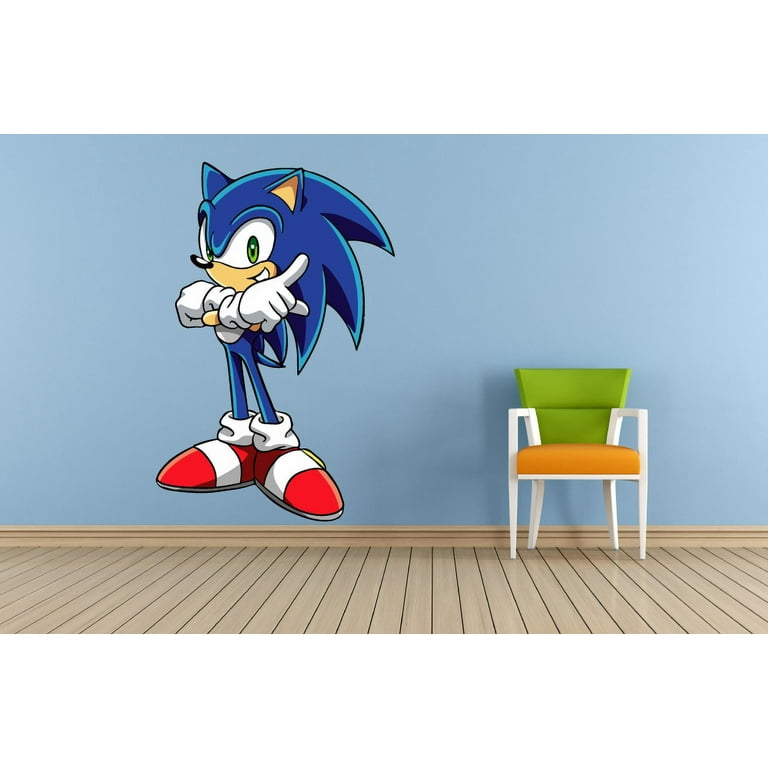Set against a light blue wall with a lighter section where light hits, this photograph showcases a sparsely furnished room. Sonic the Hedgehog, in a large and detailed portrayal, dominates the left side of the wall. Sonic's blue body, spiky hair, and green eyes are instantly recognizable, along with his signature red and white sneakers and white gloves. His arms are crossed in a confident gesture, and he points towards the upper right corner with a slight smile on his face.

The room's floor is comprised of light brown wooden boards, featuring black vertical lines that delineate each plank, and is complemented by a matching light brown wooden baseboard. On the right side of the image, next to Sonic, there is a distinctive chair with white legs and arms, an orange seat cushion, and a curvy, avocado green backrest. The minimalist setting accentuates the vibrant cartoon presence, creating an engaging and nostalgic scene.